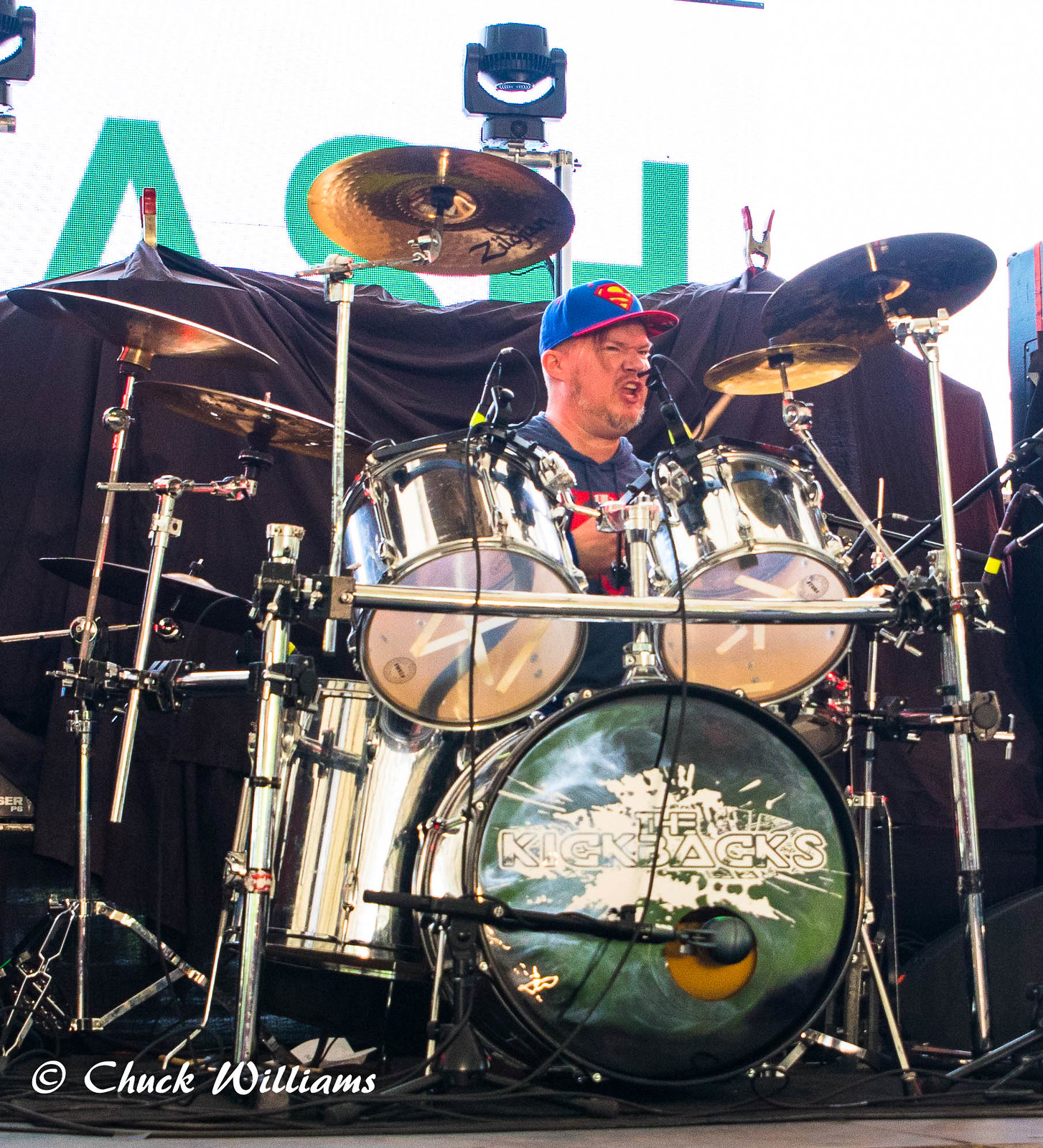In this detailed outdoor photograph by Chuck Williams, a white man is captured intensely playing the drums on stage. He sports a blue baseball cap with a red brim, emblazoned with the Superman logo, and wears a dark blue sweatshirt. His face is scrunched in a semi-frown, his mouth slightly open as if he's shouting, and his eyes squinting, suggesting a moment of high concentration or emotion. The drum set before him is extensive, primarily featuring gold-colored drums, with the large bass drum prominently bearing the words "The Kickbacks" in white lettering on a dark greenish-black surface.

The man is partially obscured by the drum set, with only his upper body visible, as the photo appears to be taken from a lower angle. To the left, at the bottom, the photograph carries a copyright notice in white text that reads "© Chuck Williams." The stage setting includes a black tarp-like curtain and numerous cables strewn about, hinting at the intricacies of the musical performance. Behind the black covering, a white wall can be seen with green letters, partially spelling out "A.S.H," along with a mounted speaker. The overall scene is a snapshot of a passionate drummer immersed in his musical element.